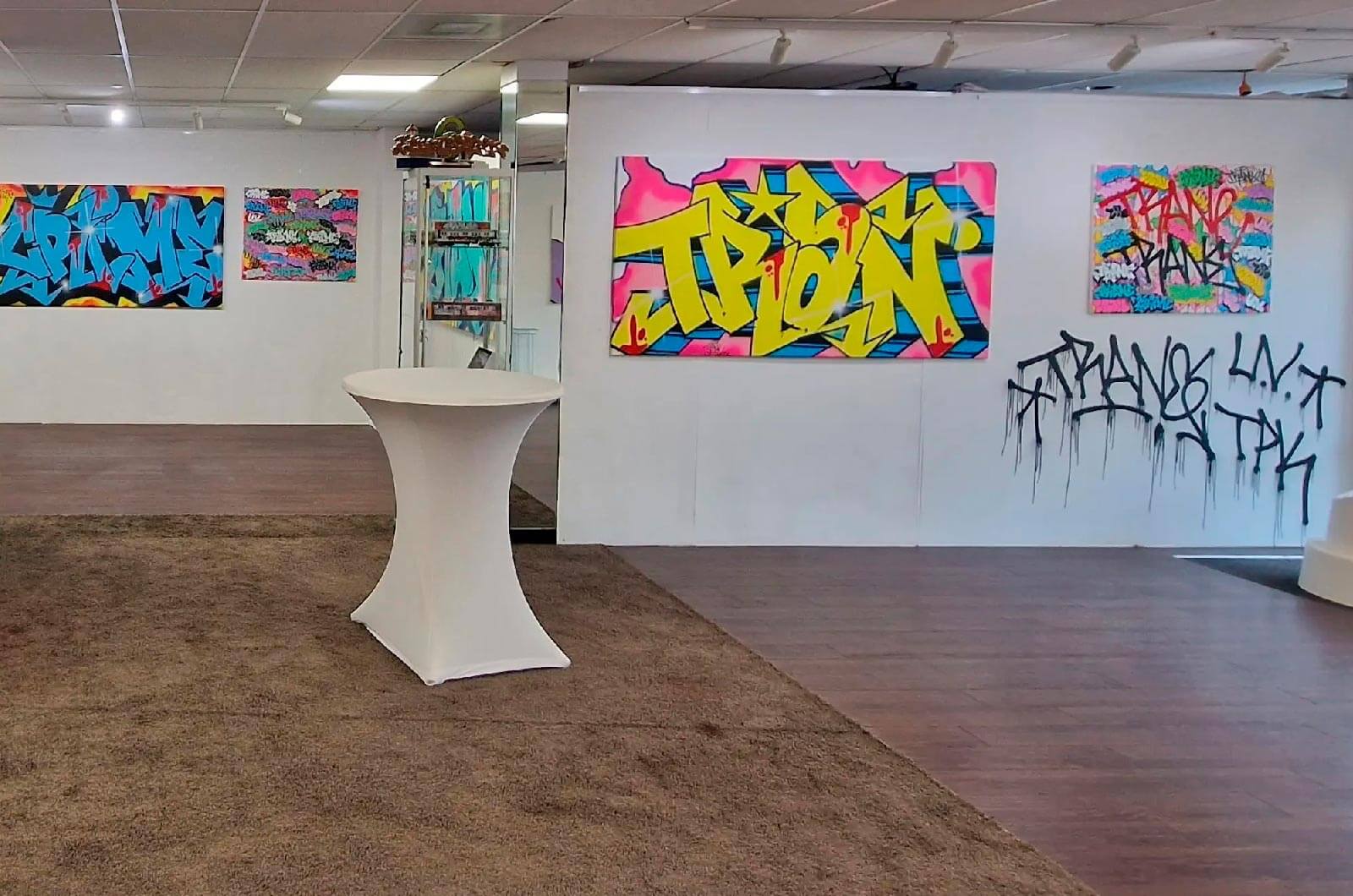The photo captures a medium-sized art gallery featuring a collection of graffiti-style art. The room is characterized by white walls and a standard white drop ceiling, creating a clean backdrop for the vibrant artwork. The right-hand side of the gallery showcases a striking piece of graffiti with a pink background and yellow lettering accented with blue and black shading. On the left-hand side, there is more graffiti art displaying blue letters on a yellow background. In the middle of the wooden-floored gallery, which also includes a carpeted section, there is a curious white pedestal with nothing on it, flanked by one or two display cases. The overall interior is brightly lit, emphasizing the bold colors—blue, yellow, pink, and black—used in the graffiti art, some of which looks like additional layers of spray paint were added. The space is a fusion of structured gallery aesthetics and the raw, expressive nature of graffiti.